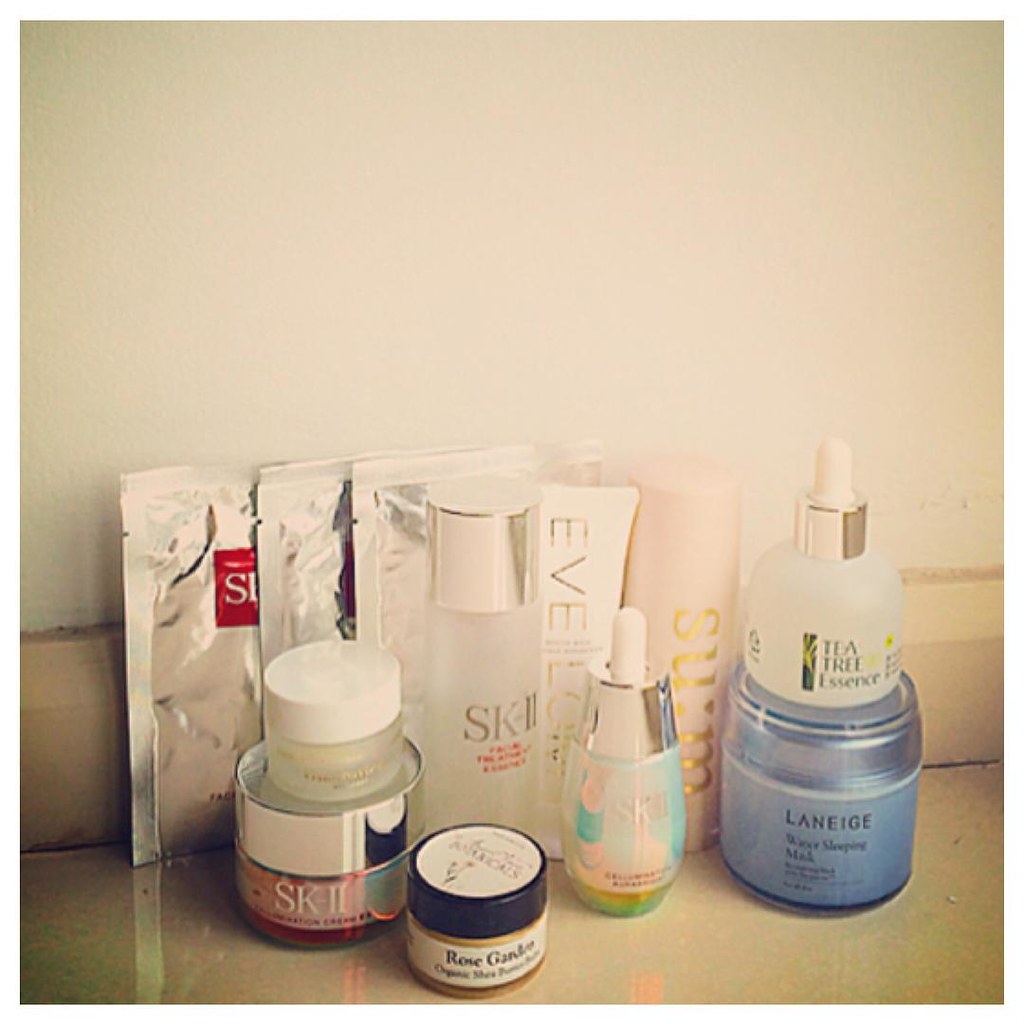The image features an off-white countertop with a splash board area running diagonally from left to right, slightly raised towards the right. Above the splash board is a white wall aligned horizontally. Various pouches, bottles, and spray bottles of cosmetics or skincare products are displayed across the lower part of the center of the image. 

To the far left, three or four foil pouches stand upright, leaning against the wall. The leftmost pouch has a visible red square on its left side. In front of these pouches, three jars of different sizes and colors (black and white, pink with a silver top, and one with a white lid) are neatly arranged.

Behind these jars, an opaque plastic bottle with a white lid is visible. To its right, a white tube with partially visible text reading "EVE" runs vertically. Next to the white tube is a slightly pink-colored tube adorned with gold lettering. Further right, a blue glass jar labeled "Laneige" in black text is seen, with a small white bottle stacked on top, labeled "Tea Tree."